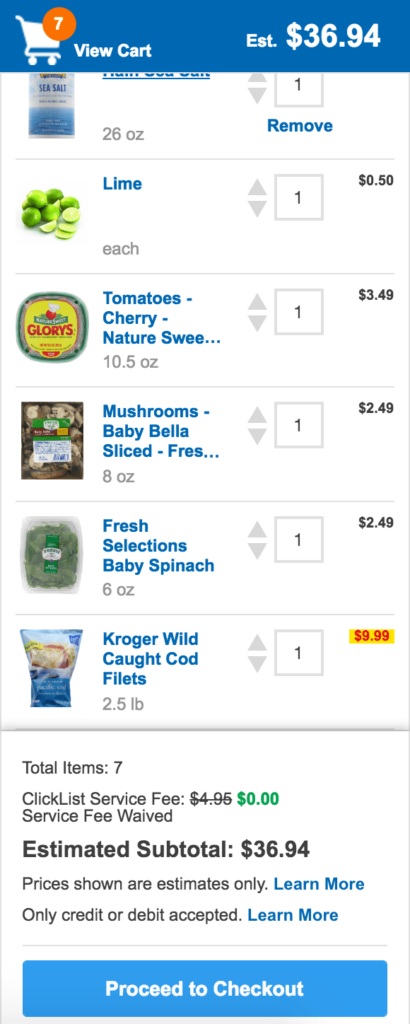The image depicts a shopping cart interface with a blue background at the top. On the top left, a white cart icon indicates "View Cart" with a number "7," signifying there are 7 items in the cart. On the top right, the total estimated price is displayed as $36.94.

In the center of the page, the background turns white, showcasing a selection of groceries. Each product has its picture on the left side and its name in blue text beside it. The items listed include:
- Green limes priced at $0.50 each.
- Nature cherry tomatoes priced at $3.49.
- Sliced baby bella mushrooms, brown and white, priced at $2.49.
- Fresh Selection baby spinach, green, priced at $2.49.
- Wild-caught croaker fillets, priced at $9.99. The price is highlighted in red against a yellow background.

At the bottom, a summary section details the cart information: "Total Items: 7," with a "Service Fee" originally listed at $4.95 but scratched out and shown as "$0.00" in green, indicating that the service fee is waived. The estimated subtotal remains at $36.94, with a note that the prices shown are only estimates and payment can only be made using a credit or debit card. The page concludes with a blue "Proceed to Checkout" button in white text.